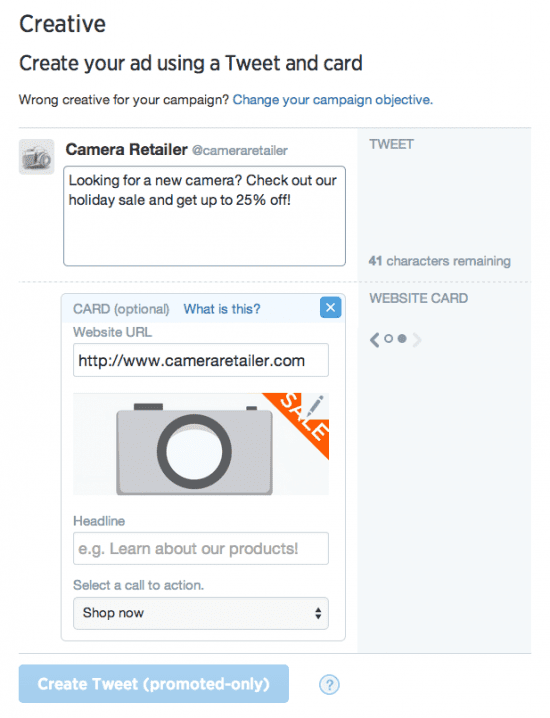This rectangular screenshot captures a user interface for creating an advertisement using a tweet and a card. The upper left corner of the image features a bold black title that reads "Creative." Just below, a subheading provides further instructions: "Create your ad using a tweet and card."

The main panel of the interface is organized and clearly labeled, starting with "Camera Retailer" in bold black font. Below this heading is a large, rectangular text field with a white background and black text, displaying the message: "Looking for a new camera? Check out our holiday sale and get up to 25% off."

Next, there's an optional section for adding a card, indicated by the word "Optional" in light gray text. Beneath this is a text field designed for a website URL. This elongated, rectangular field has a white background with black text, bearing the URL: "http://www.cameraretailer.com."

Further down, a large camera icon is prominently displayed. The base of the icon is light gray, while the lens and a few buttons on the top are in dark gray.

Following the icon, there is a line for the headline indicated in light gray text. Under this, another long, rectangular text field with a white background and gray writing offers an example headline: "e.g. Learn about our products."

The final element in the panel is a drop-down menu for selecting a call-to-action, labeled "Select a call to action." This menu has a light gray background and black text displaying the option "Shop Now."